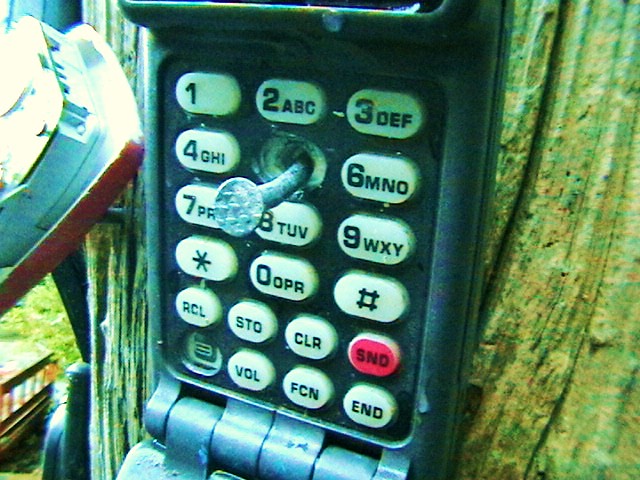In this outdoor photo, a vintage flip phone, reminiscent of early mobile devices, is prominently displayed nailed to a weathered wooden post, with grass faintly visible in the background. The phone is pinned open through the number 5 key, which is conspicuously absent, revealing a substantial metal nail driven through it. Other identified keys include numerical keys 1 through 9, with associated letters, and several function keys such as RCL, STO, CLR, VOL, FCN, and a red SND button, among others. While the flip phone shows signs of aging, it remains largely intact apart from one button on the bottom left corner that exposes its circuitry. Adjacent to the phone, though somewhat washed out in the left corner of the image, appears to be an additional device, potentially some type of electrical equipment or light, also affixed to the post with a protruding nail.